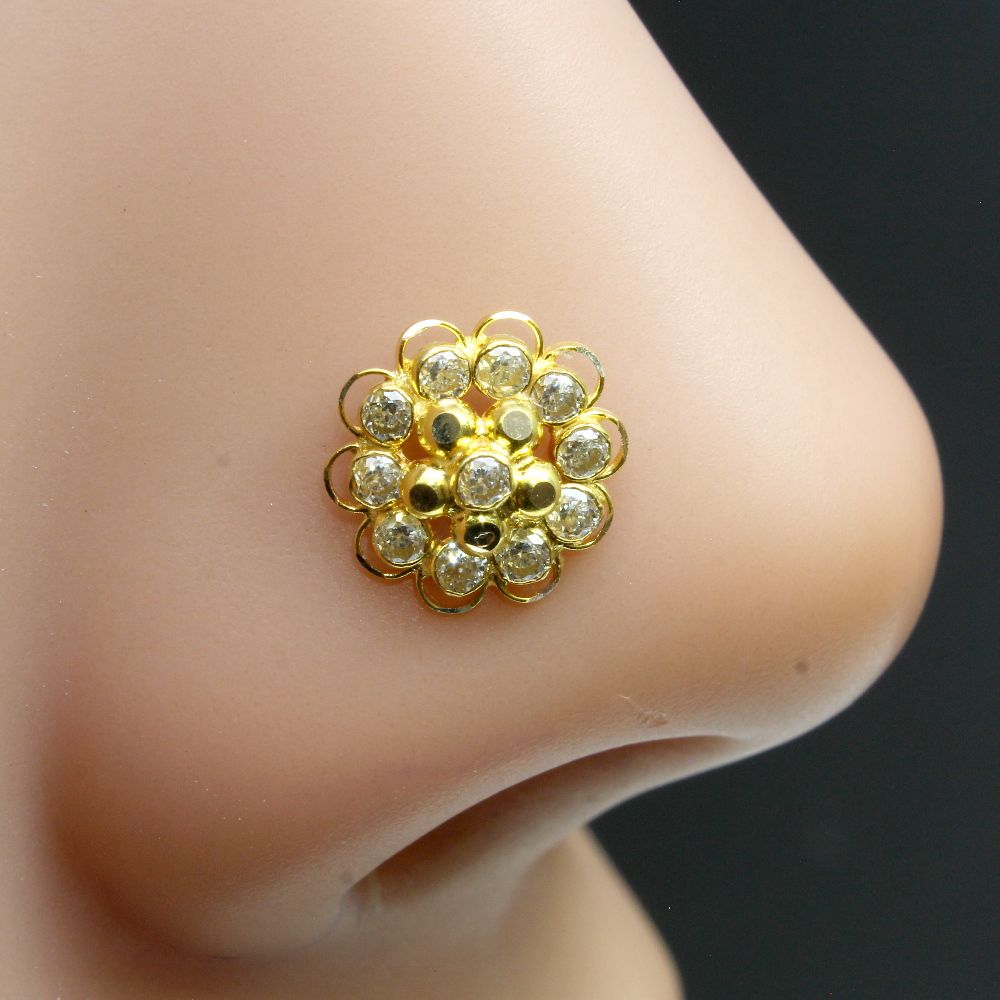The image is a close-up, side view of the lower part of a very smooth, light-skinned nose, adorned with an ornate gold nose piercing. The backdrop is a stark, dark gray which makes the details of the nose and jewelry stand out prominently. The piercing is shaped like a flower, featuring an intricate arrangement of gold loops and circular patterns. It includes ten circular diamonds denoting the edges of the petals, with five smaller diamonds forming the inner part of the flower, all culminating in a larger central diamond. There are slight imperfections observable on the skin, such as a small skin tag and a mole near the nostril, with hints of redness toward the base of the nose. The nose jewelry appears to be crafted from gold, accented with diamonds, and there are areas of shadowing, possibly contributing to the perception of additional dark elements within the ornament. The overall appearance is highly detailed and visually striking, suggesting refined craftsmanship.